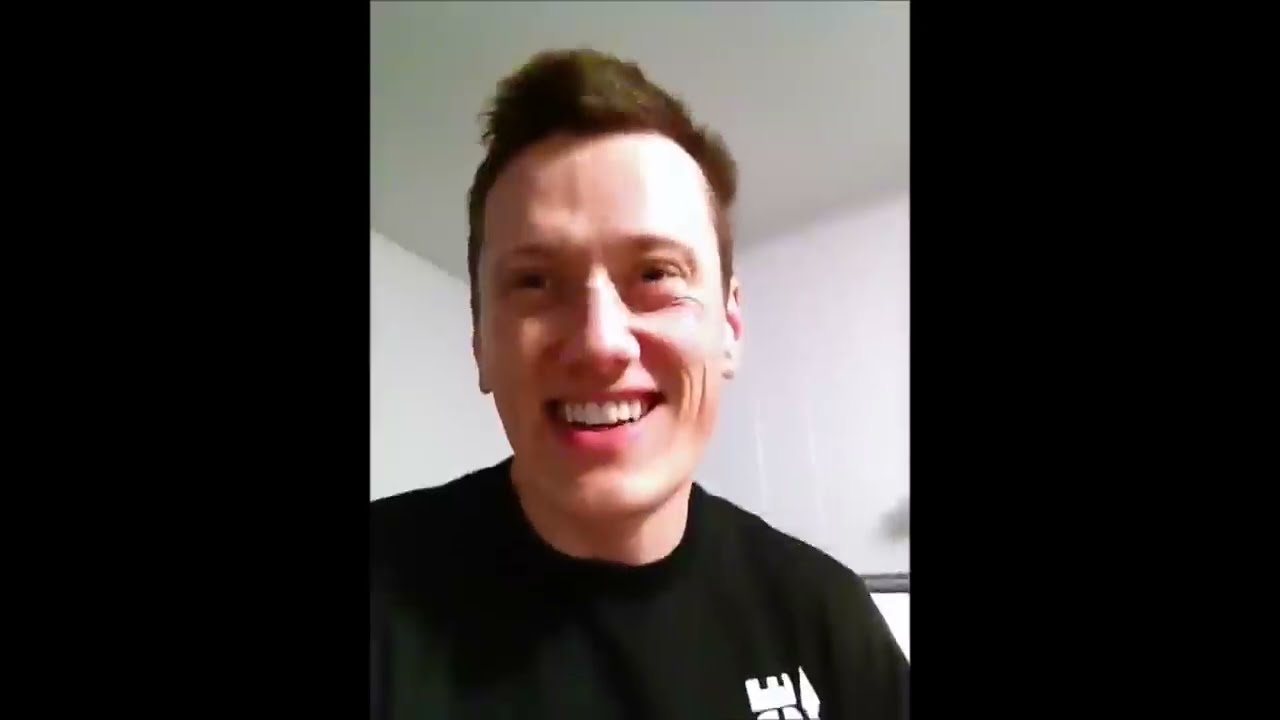The image features a close-up photograph of a young Caucasian man in his early to mid-20s, looking slightly to his left with an expression of surprise. His wide-open hazel eyes and mouth, parted as if he's speaking or gasping, convey a sense of shock. His short, thick dark hair, sticking up a little at the front, complements his clean-shaven face. His forehead is creased with a few wrinkles due to his raised eyebrows.

The man is wearing a black t-shirt, but only his shoulders are visible in the vertically cropped photo. The background shows the plain white ceiling and walls of a room, with a slight shadow at the corner where the wall meets the ceiling. The image itself is slightly blurry as if taken mid-motion, and it is framed by black borders on the left and right sides. A faint pinkish tone is noticeable on his cheeks and lips, adding to the vividness of his surprised expression.